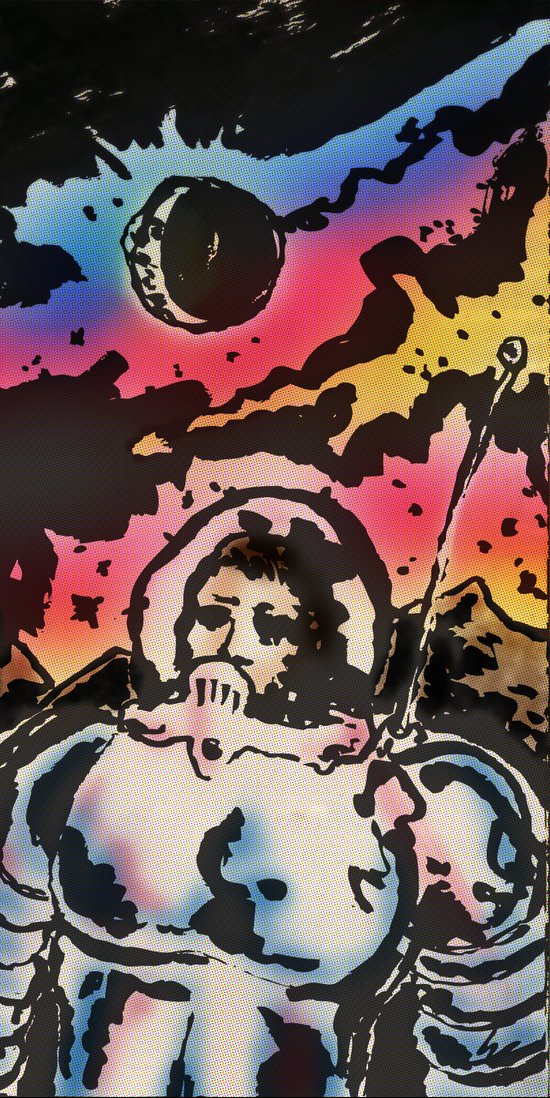This is a detailed digital drawing showcasing an astronaut, clad in a predominantly white space suit accented with blue, pink, and detailed black lines. The astronaut, who appears to be a woman, is depicted with a glass dome helmet, through which her face is visible. An antenna protrudes from the left shoulder of the suit. There are intricate robotic-like horizontal lines running across the arms and a chest plate with an outward indentation. The background is a vibrant alien sky filled with blue, pink, and yellow clouds, and a black, crescent-like moon or meteor punctuates the scene. Above, the sky transitions through various colors, including black, blue, red, yellow, and brown, with an impressionistic pattern. Dominating the background is a dramatic volcano, spewing rocks, debris, and smoke into the air, adding to the otherworldly atmosphere of the scene.